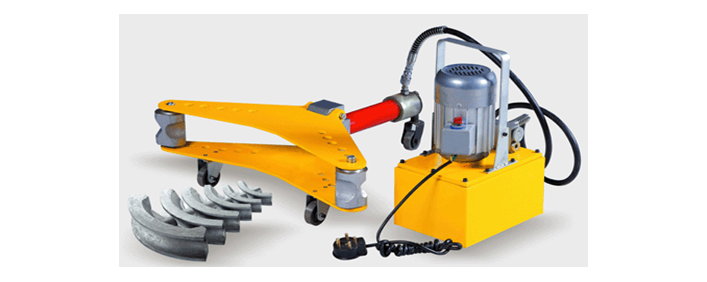The photograph is a high-quality product image of an industrial electronic machine, captured on a solid white background and surface, ideal for online listings, catalogs, or commercial websites. The machinery is comprised of several distinct components: the right-hand side features a robust, rectangular yellow metal box with black bolts securing its lid. Above this yellow box is a silver cylindrical motor equipped with vents and a silver handle. Extending from the front of the box is a black electrical plug with a three-prong end, and a separate black tube connecting to another component.

This additional section is characterized by a horizontal red bar supporting the primary elements. At the end of this bar is a set of two boomerang-shaped yellow plastic pieces, held together by gray cylinders. These plastic elements connect to curved metal platings at the lower left, which extend in varying lengths and widths. The machine's added mobility is provided by several small wheels underneath. Together, these components create a complex machinery system, designed for specialized industrial use.